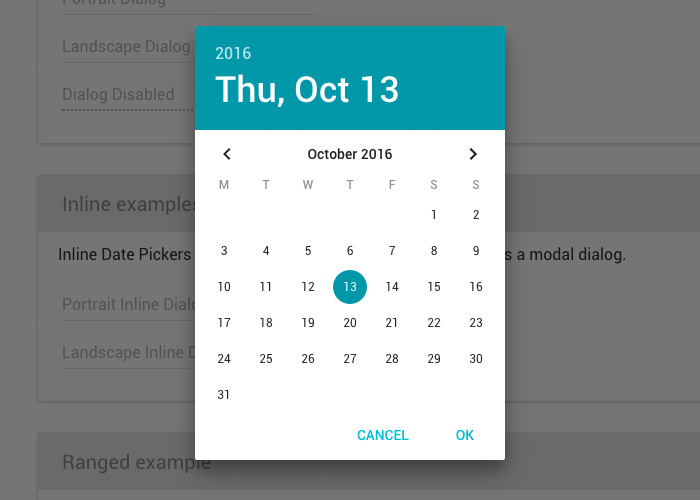The image depicts a user interface with several overlapping elements. The background is grayed out, providing contrast to the various dialog boxes layered on top. At the highest level, there is a title labeled "Landscape Dialog." Beneath it, a series of labels read: "Dialog Disabled," "Inline Examples," and "Inline Data Pickers." Partially obscured by these elements, additional text indicates "SA Model Dialog," "Portrait Inline Dial," "Landscape Inline D," and "Range Examples."

Dominating the foreground is a calendar interface displaying the date "Thursday, October 13th, 2016," highlighted within a blue rectangle banner. Below the banner, the calendar is arranged in a standard format with the days of the week noted as "M, T, W, T, F, S, S" representing Monday through Sunday. The entire month of October 2016 is visible, starting from the 1st and ending with the 31st. The 13th is marked with a distinct circular bubble, denoting a current selection or an important event.

Flanking the bottom of the calendar are two action buttons: "Cancel" on the left and "OK" on the right, allowing the user to either dismiss the calendar or confirm their selection.